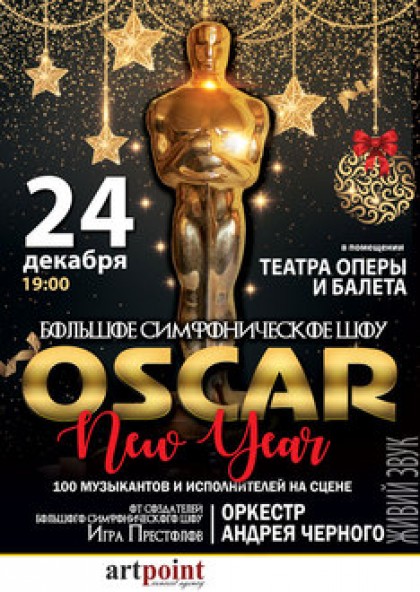The image is a full-color, vertical rectangular advertisement for the "Oscar New Year" event, featuring Eastern European, likely Cyrillic, text. At its center stands a prominent gold Oscar trophy with the number "24" in white to the left. Draped behind are elegant gold stars and decorations, including a gold and black Christmas ornament with a red ribbon, creating a festive atmosphere. The word "Oscar" appears in bold, shaded gold uppercase letters across the bottom of the trophy, while "New Year" is styled in red script atop the word "Oscar". The time "1900:00" is noted, indicating the event's schedule. At the very bottom, the designer's mark reads "Art Point," with "Art" in black and "Point" in red, accompanied by a black dot, all presented in a modern style.